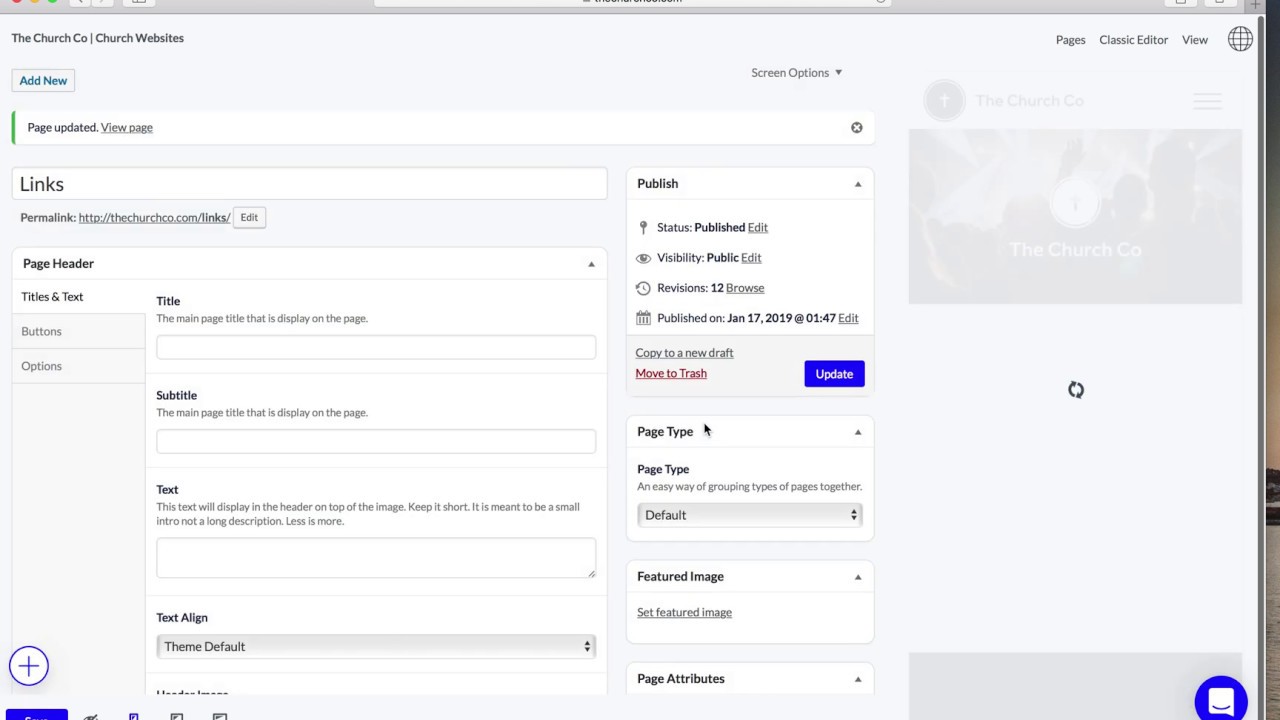This screenshot captures a portion of a website’s content management system, specifically dedicated to church website development. In the upper left-hand corner, the text reads “The Church Company / Church Websites.” Below this heading, there is a blue "Add New" button housed within a white box. 

On the right side of the interface, options to access "Pages" and "Classic Editor View" are available. Central screen options include features such as "Page updated" and "View Page," indicating updates and review functionalities.

The middle section lists various elements like "Links," which offer page headers, titles, and text specifications. It includes buttons and settings for adjusting titles, satellite options, and text alignment. Additionally, on the right side of the interface, a column begins with "Publish." This column details the publishing status, visibility (public), and revision history (12 revisions), along with options to edit these attributes. It displays the publication date and has further controls for moving the page to trash or updating the page type.

Beneath page attributes, there are customizable sections such as "Featured Image" and a default button under "Page Type." The comprehensive array of options necessitates familiarity with various computer terminologies for effective navigation and operation.

Interestingly, behind this web page, there is a semi-transparent image that appears to be a credit card adorned with floral patterns, suggesting a visually appealing design interface interwoven with the technical elements.